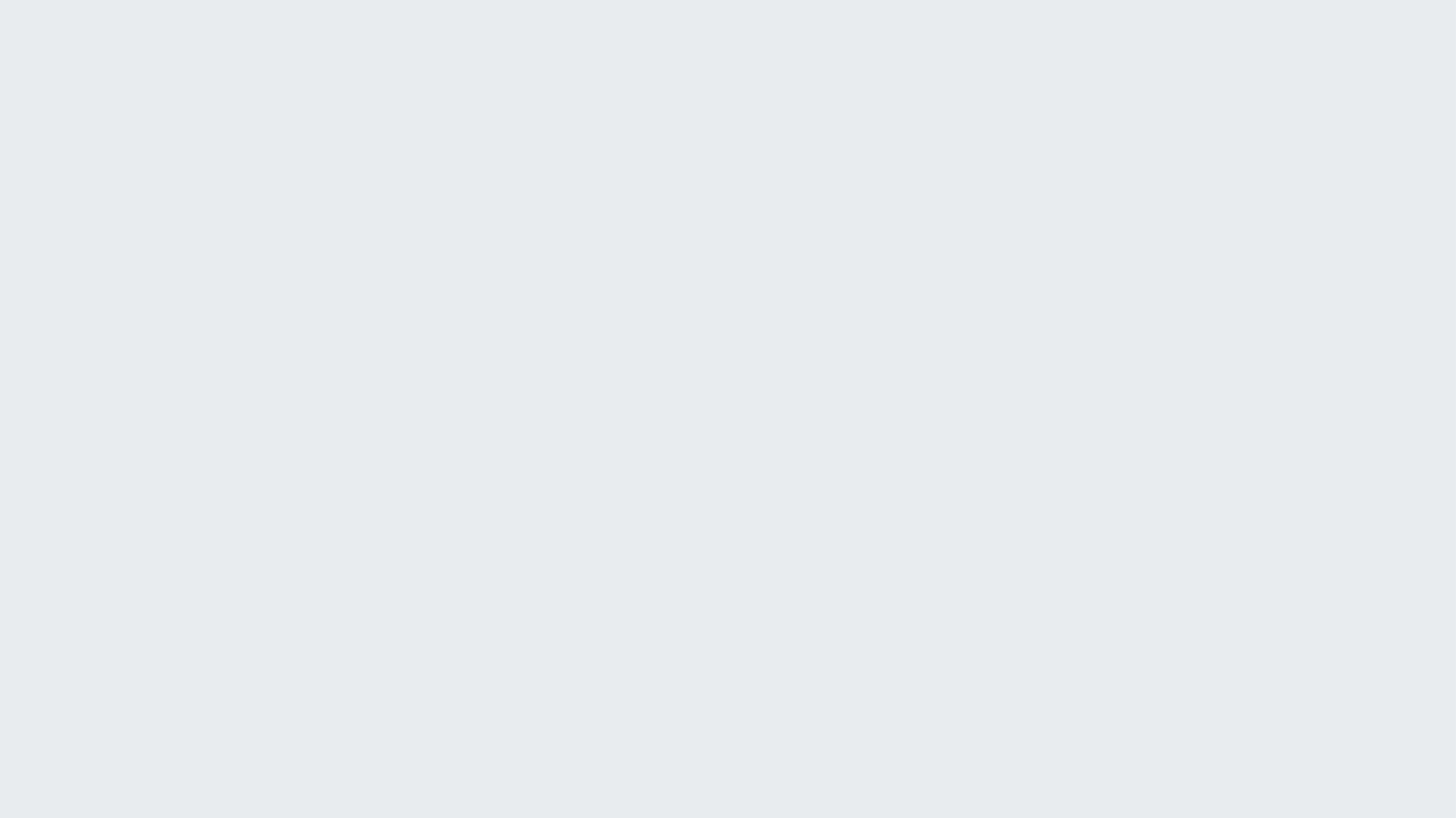A plain, featureless rectangle is displayed in landscape orientation, offering no discernible text, objects, or background details. The rectangle's surface is entirely devoid of color, style, or any form of decoration, resembling a blank screen or possibly a gray piece of construction paper. Its proportions suggest that if divided in half, it would form nearly two perfect squares. There is neither an outline nor a frame to define its edges, reinforcing its stark emptiness. This unremarkable image stands as a testament to minimalism and the absence of visual content.